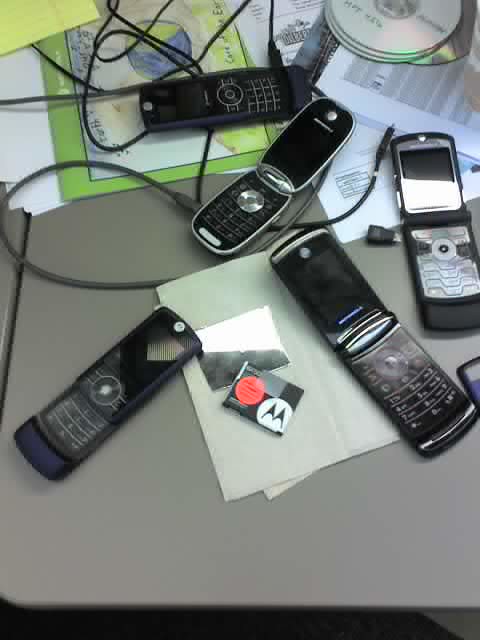This image captures a collection of five dated flip phones, primarily in black with silver accents, arranged haphazardly on a gray desk. The phones, identified as older models possibly including a Motorola device, are accompanied by a distinctive Motorola logo on one piece of paper. The devices are intermixed with various black charging cords, CDs, and a scattering of papers. Notably, the papers include a lime green sheet and a child-colored image. The desk is cluttered, featuring additional elements such as an item with "AA" in a red circle and other unidentifiable text. Overall, the scene evokes a sense of nostalgia, emphasizing obsolete technology amid everyday desk clutter.